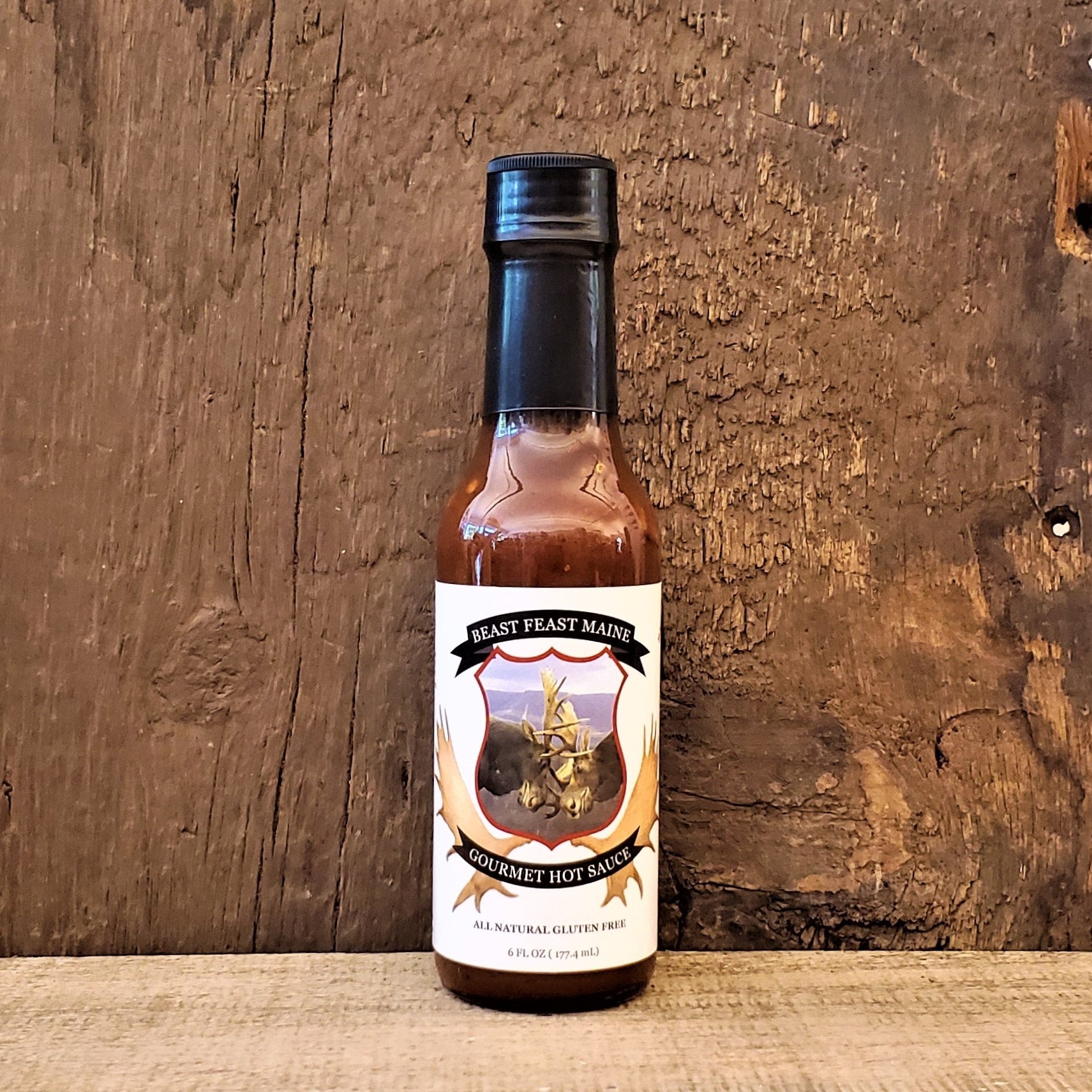The image is a close-up of a small glass bottle of hot sauce labeled "Beast Feast Maine Gourmet Hot Sauce," which is all-natural and gluten-free. The bottle, containing a reddish-brown hot sauce, has a black protective seal around its neck and a white label displaying a logo shaped like a badge. The logo features an illustration of two rams locking horns. The bottle is placed on a light brown wooden surface, set against a weathered, dark brown wooden backdrop, possibly a tree with visible cracks and wear.